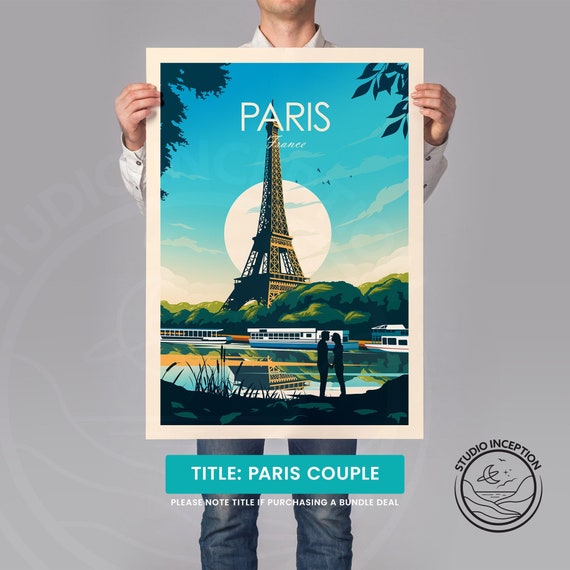A man, visible from his chin down to below his knees, is holding a meticulously detailed advertisement poster for Paris in both hands. He is dressed in a white collared shirt. The poster, framed by a white border, features a vivid blue sky with trees on either side. Central on the poster is the iconic Eiffel Tower, flanked by greenery, buildings, and a river, all rendered in a hand-drawn style. Below the scenic illustration, a couple's silhouette stands in a garden-like setting, capturing a romantic moment. The poster's bottom half contains text: a blue border with the white title “Paris Couple”, and a notice below it, "Please note if purchasing a bundle deal." In the bottom right corner, a circular logo with a spaceship and the text "Studio Inception" in black is prominently displayed, indicating the poster's creator. The backdrop of the image is a uniform grey, ensuring the vibrant colors and illustrative details of the poster stand out clearly.